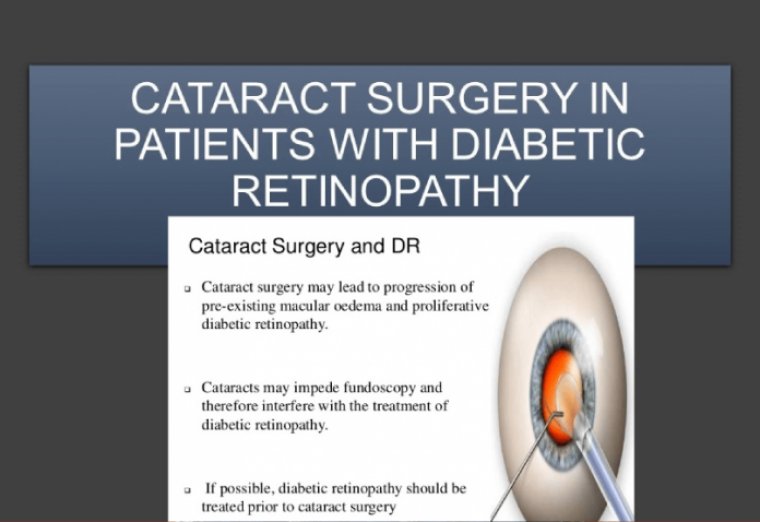The image, rectangular in shape and resembling a page from a medical textbook or doctor's magazine, measures approximately six inches wide by four inches high. It features a dark gray, almost black, background at the top. Inserted from the left and right edges by about a quarter of an inch and descending from the top border by about half an inch is a horizontally oriented, dark blue rectangle with a black outline. The rectangle contains three rows of white capital letters that read "CATARACT SURGERY IN PATIENTS WITH DIABETIC RETINOPATHY."

Below this, a white square extends downward, containing a detailed diagram of an eyeball with surgical tools interacting with it. The eyeball is depicted with a blue iris and an orange center, highlighting where the lens is being removed. To the left of this diagram, the text "CATARACT SURGERY IN DR" is printed in blue.

Beneath this, there are three bullet points providing important information:
1. "Cataract surgery may lead to progression of pre-existing macular edema and proliferative diabetic retinopathy."
2. "Cataracts may impede fundoscopy and therefore interfere with the treatment of diabetic retinopathy."
3. "If possible, diabetic retinopathy should be treated prior to cataract surgery."

This informative and visually detailed image emphasizes the complexities and considerations of performing cataract surgery on patients with diabetic retinopathy.